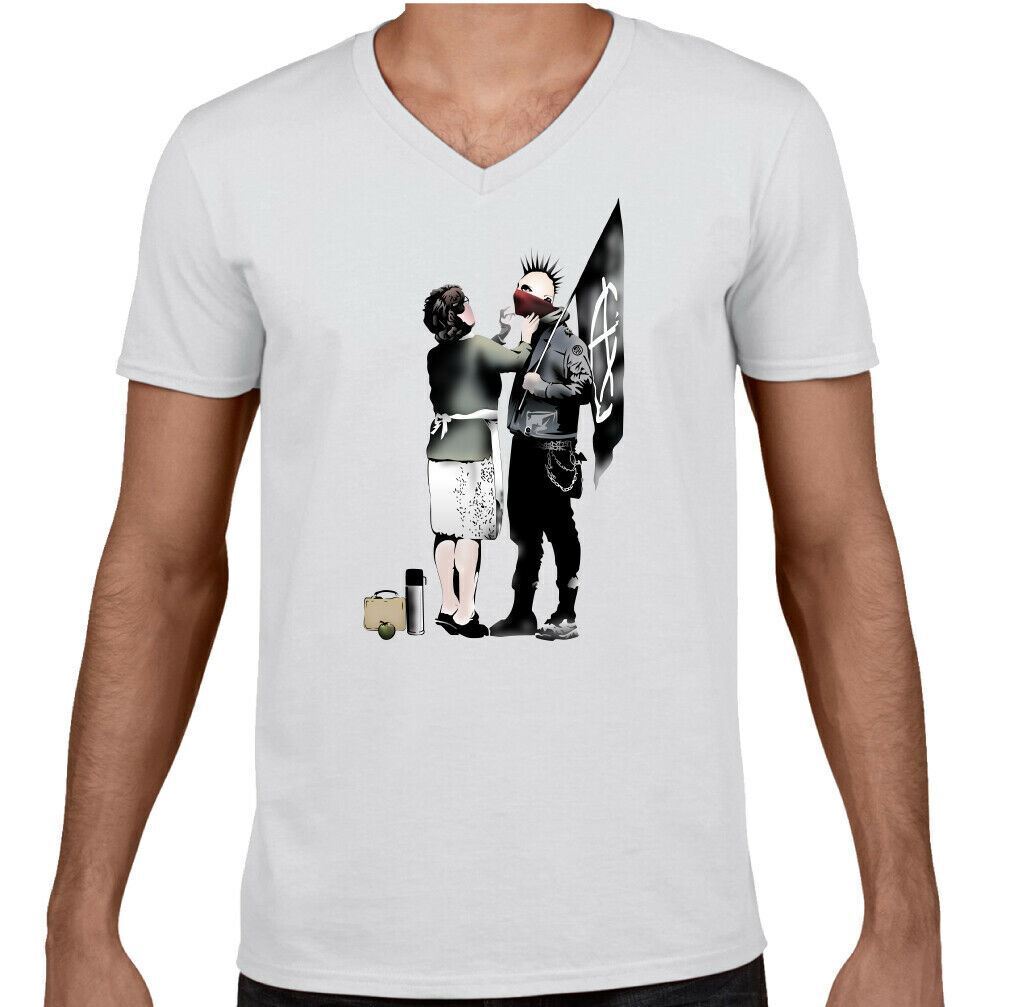The image depicts a man wearing a white t-shirt emblazoned with an eclectic and humorous graphic. The graphic features a punk anarchist, identifiable by his spiked black mohawk, red bandana covering his face, black leather jacket, and black pants adorned with chains. He is holding a black flag emblazoned with the anarchist symbol. Standing in front of him is a woman dressed in stereotypical 1950s housewife attire: a dark green blouse, skirt, heels, and an apron. Her hair is tied back as she tenderly adjusts the anarchist's bandana. On the ground beside her, there is a packed lunch consisting of a tan lunchbox, a green apple, and a thermos, suggesting she is preparing him for his day. The graphic appears to be poorly photoshopped onto the white v-neck shirt the man is wearing, reminiscent of the type of images commonly seen on online retail sites.